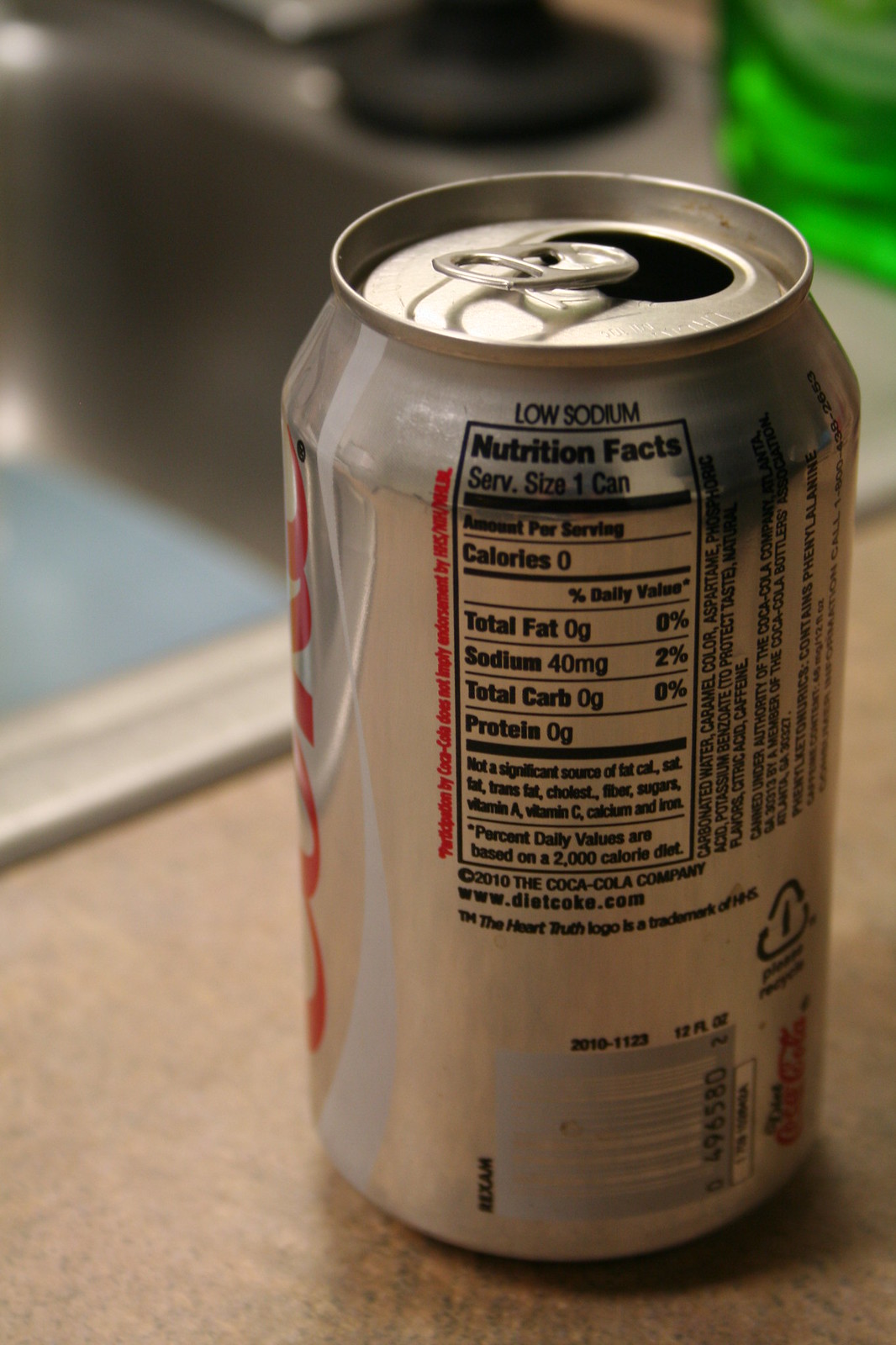The image features a silver can of Coca-Cola positioned on a brown counter. In the lower right-hand corner, the can is turned such that the Nutrition Facts panel and the low sodium label are visible, with text printed in black ink. The iconic red Coca-Cola logo is partially seen on the left side of the can. Below the Nutrition Facts, near the bottom right, there is a recycle symbol. The center bottom of the can displays a white or silver EPC code. The can is open at the top.

In the upper left corner of the image, there is a blurry, square object with a white border and blue center, making it indiscernible. Behind the can, situated in the upper right corner, there appears to be the base of a bottle of green dishwashing liquid, suggesting that to the left of the can is a kitchen sink. The overall setting indicates a typical kitchen environment.